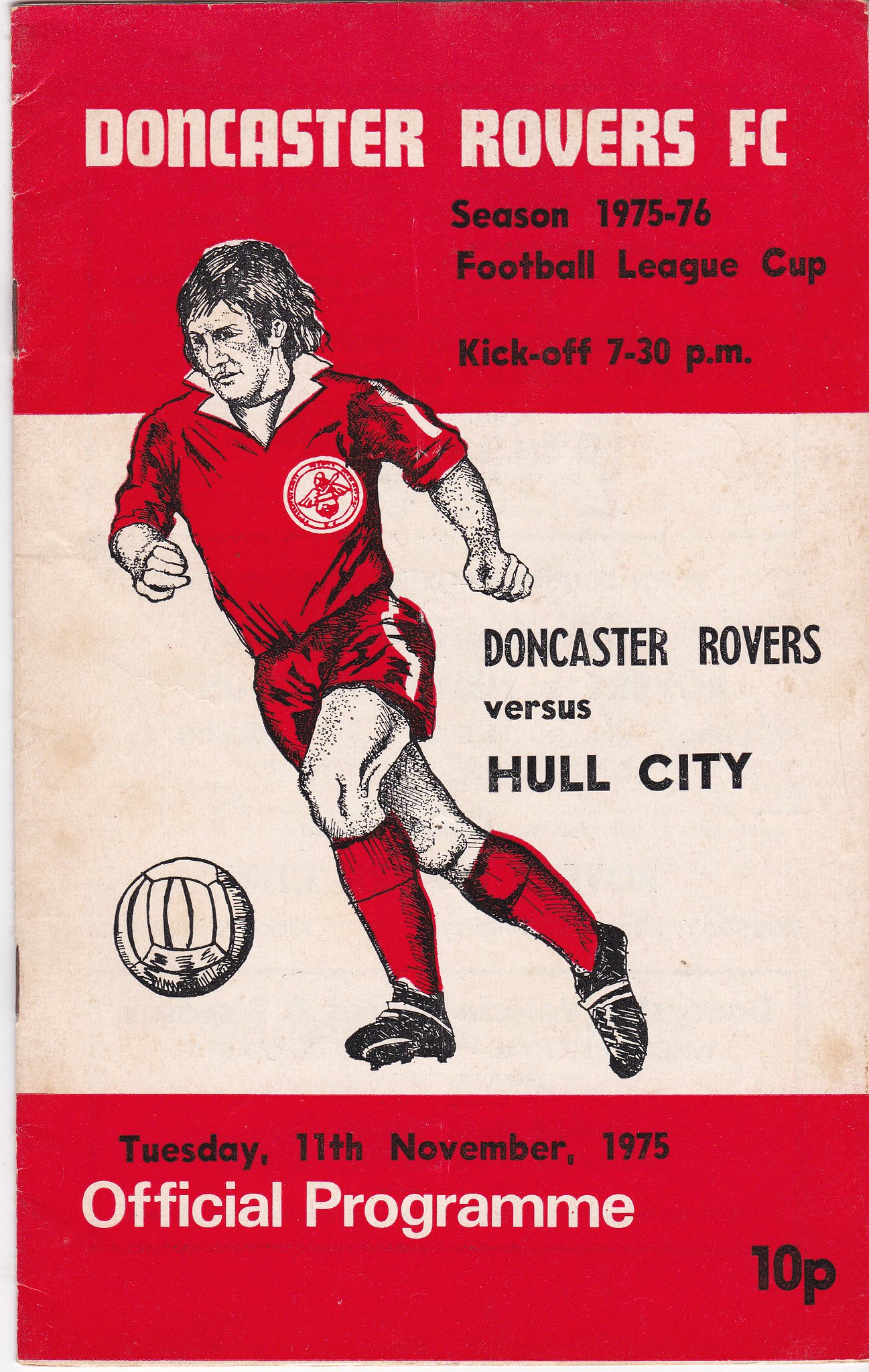The image is the cover of an official program for a football match. The cover has prominent red sections at the top and bottom. At the top, the text "Doncaster Rovers FC" is written in white, followed by the details "Season 1975-1976 Football League Cup" and "Kick-off 7.30 PM" in black. Below this, against a white background, it says "Doncaster Rovers vs. Hull City." An illustrated player, who has medium-length, slightly unkempt hair, is central to the design, partially extending into the red upper section. The player is depicted in a red jersey with a white collar, red shorts featuring a white stripe, red socks, and black cleats. He is shown chasing a white football. At the bottom, in the red section, the text reads "Tuesday, 11th November 1975, Official Program," and at the bottom right corner, the price "10p" is printed in white.